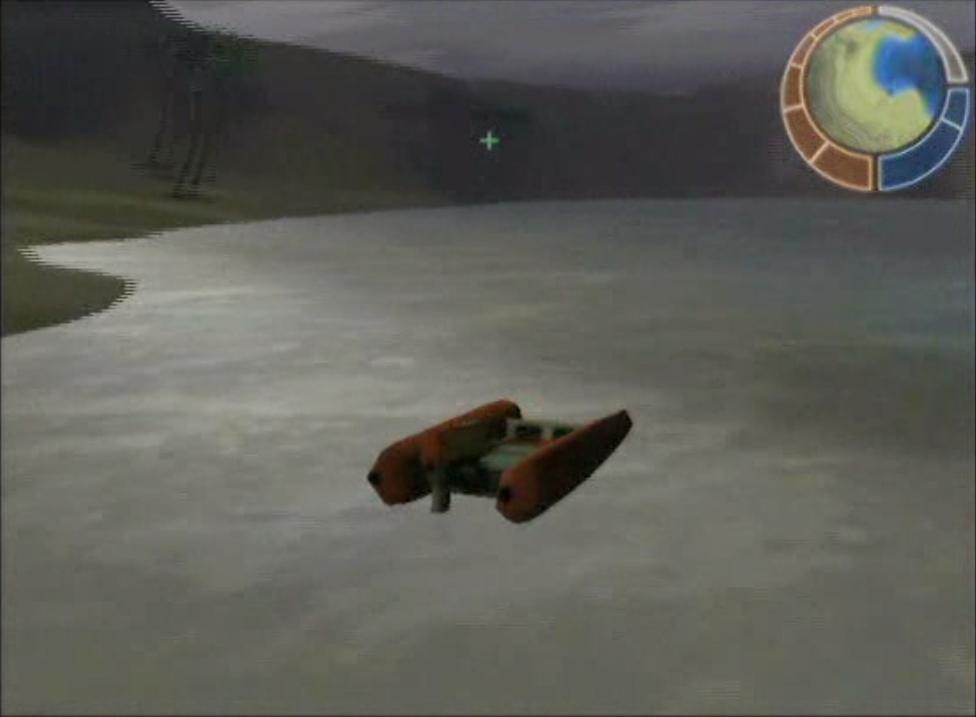The image is a widescreen screenshot from a video game depicting an overcast, hazy day on an alien planet. Covering the bottom two-thirds of the scene is a grayish expanse, likely water or ice. Above this stretches a landscape with green hills and brown-gray mountains, set beneath a solid, mostly white sky with patches of gray clouds. On the left side of the image, three trees are visible. The focus is on a craft in third person view: it features two parallel cylindrical pontoons connected by crossbars, with a rust color and traces of green. In the upper right corner of the screen, there is a multi-colored radar or map display, consisting of yellow, blue, gray, and orangey-brown segments.